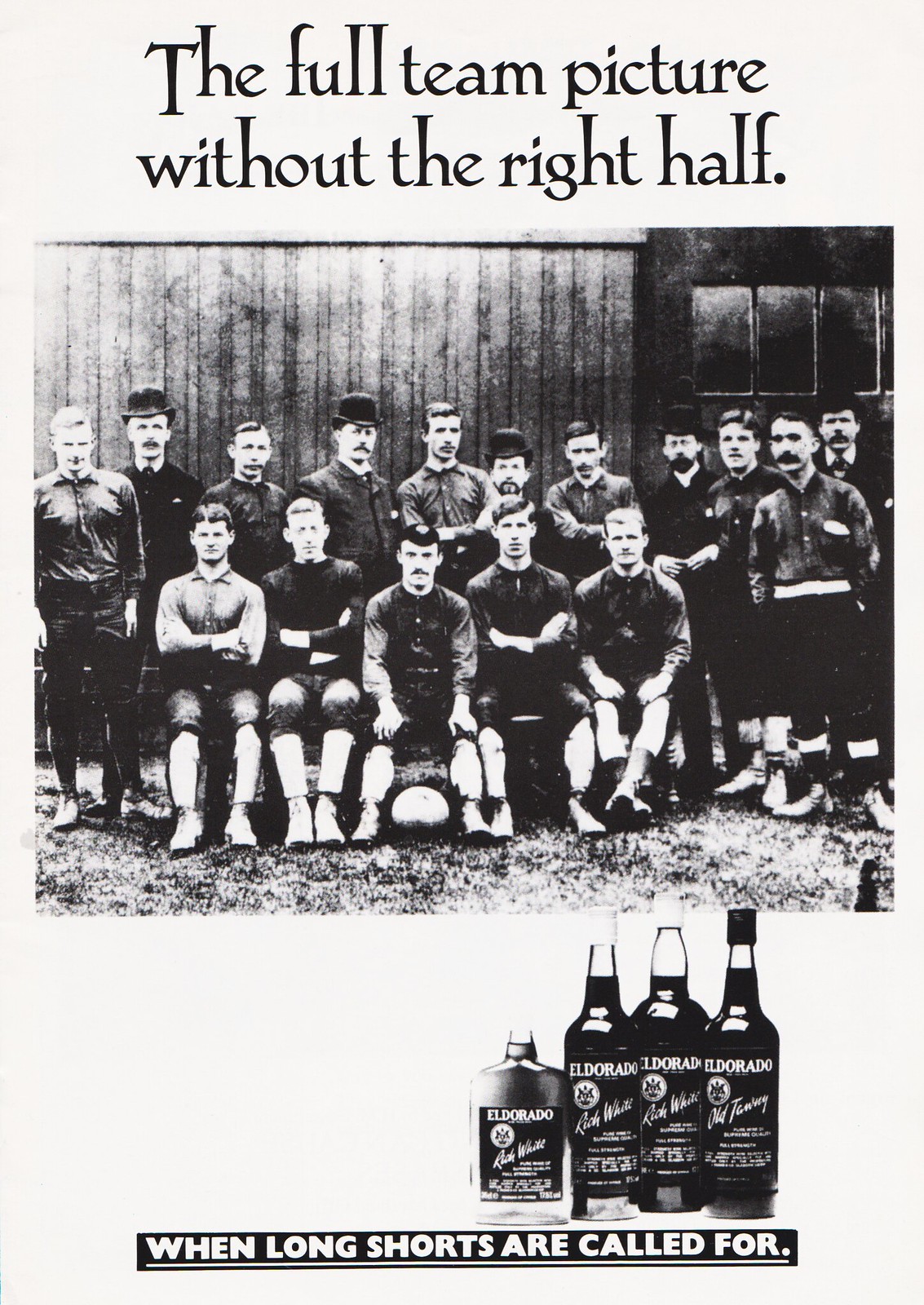This image is a vintage black-and-white advertisement, possibly from a magazine or a soccer/football club program. It features a portrait-oriented page with a white background. The headline at the top reads in black writing: "The Full Team Picture Without the Right Half." Below this, there's a half-page, landscape-oriented black-and-white photograph of a group of serious-looking men, possibly part of a soccer team. The team includes ten men standing in the back row and five seated men in the front row. Some of the seated men appear to be wearing shin guards, and one man in the center has a ball between his legs. The men are dressed in dark shirts, pants, and several are adorned with fancy hats, such as top hats. Behind the back row stands a metal building with windows visible on the right side. Below the photo is a product image featuring four bottles of El Dorado alcohol, though the specific details on the labels are not entirely readable. Below the bottles, in a horizontal black strip with white text, the slogan reads: "When Long Shorts Are Called For." The advertisement's style reflects a vintage print publication.